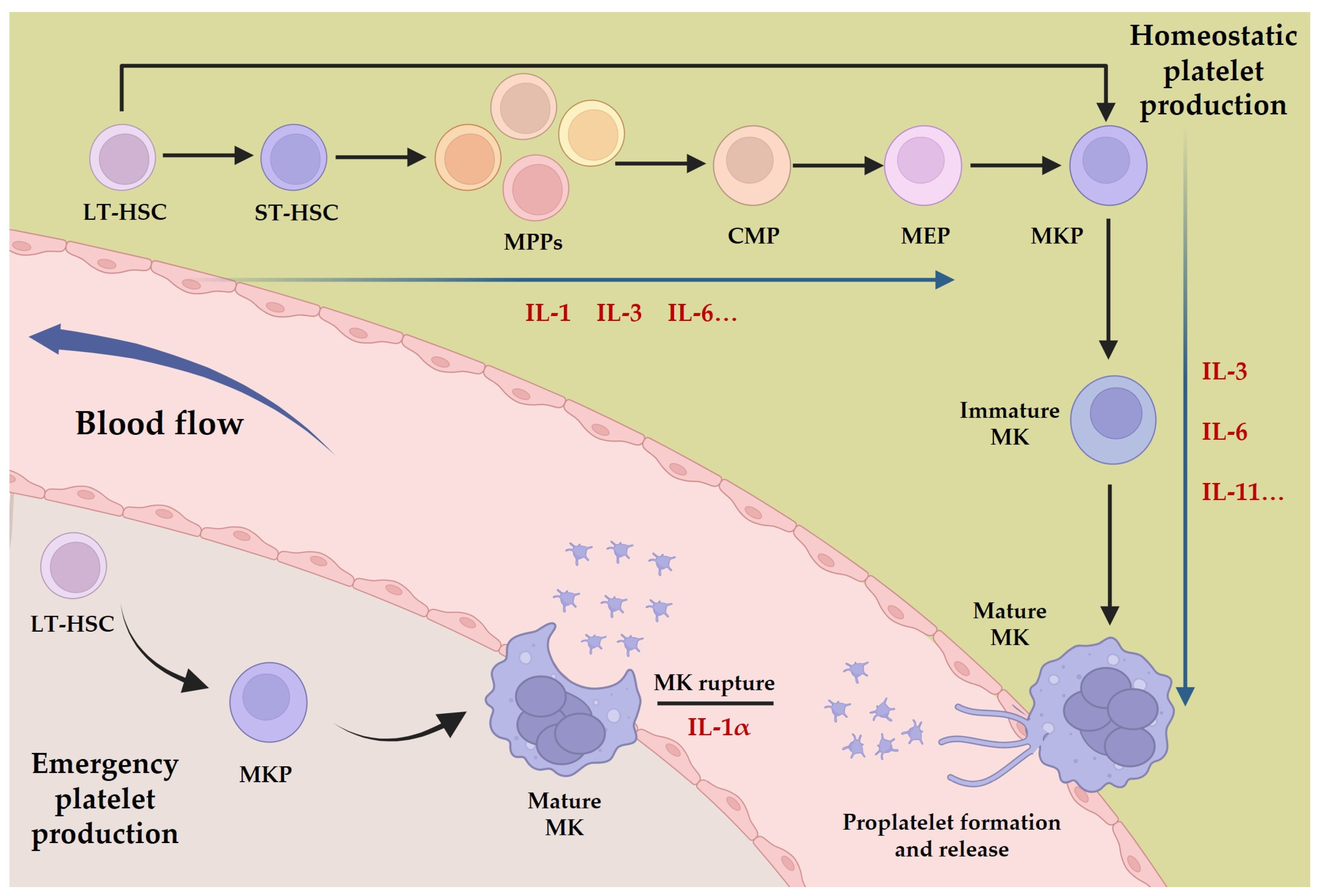This detailed graphic chart illustrates the homeostatic and emergency pathways of platelet production in the human body, likely designed for medical education purposes. It features a variety of color-coded circles, each labeled with specific abbreviations representing different stages in platelet production: LT-HSC (a purple circle), ST-HSC (a blue circle), MPPs (multiple colors including orange, brown, yellow, and pink), CMP (brown), MEP (purple), MKP (blue), immature MK (blue with wavy borders and tendrils), and mature MK (a complex structure with five internal circles). The diagram traces the process from LT-HSC to mature MK, highlighting the role of blood flow and including indicators for IL-3, IL-6, and IL-11. Additionally, it details the MK rupture process, associated with IL-1A, and a segmented portion of the image emphasizes "emergency platelet production" in the bottom left corner. This comprehensive chart combines visually distinct elements to depict the intricate steps and regulatory mechanisms involved in platelet production.